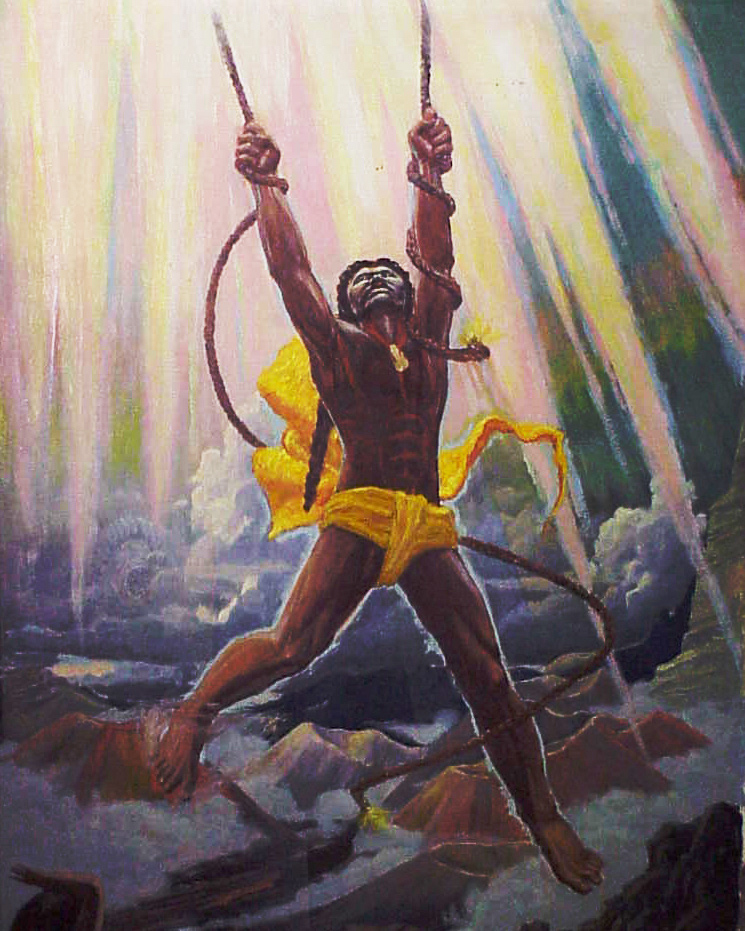This painting depicts a muscular, dark-skinned African man suspended in mid-air, his body stretched and elevated against a dramatic backdrop of mountainous regions and a vibrant, multi-colored sky. His arms are outstretched, each hand gripping a rope that ascends towards a radiant light source at the top of the composition, casting bright yellow light with pink highlights. The man, adorned with very long braided hair, gazes upward, his expression intense and focused. He wears a yellow or golden sash tied around his waist, flowing gracefully behind him, and a red necklace featuring a gold medallion. The ropes, draped around his wrists and forearms, coil around his body—one winding around his leg—and each ends in a decorative yellow tassel. His legs appear elevated as if hovering or stepping onto a cloud, enhancing the mystical and powerful aura of the scene, suggesting that he might be pulling the sky or the sun downward. The interplay of the vibrant sky and the dramatic lighting enhances the surreal and dynamic nature of the artwork.